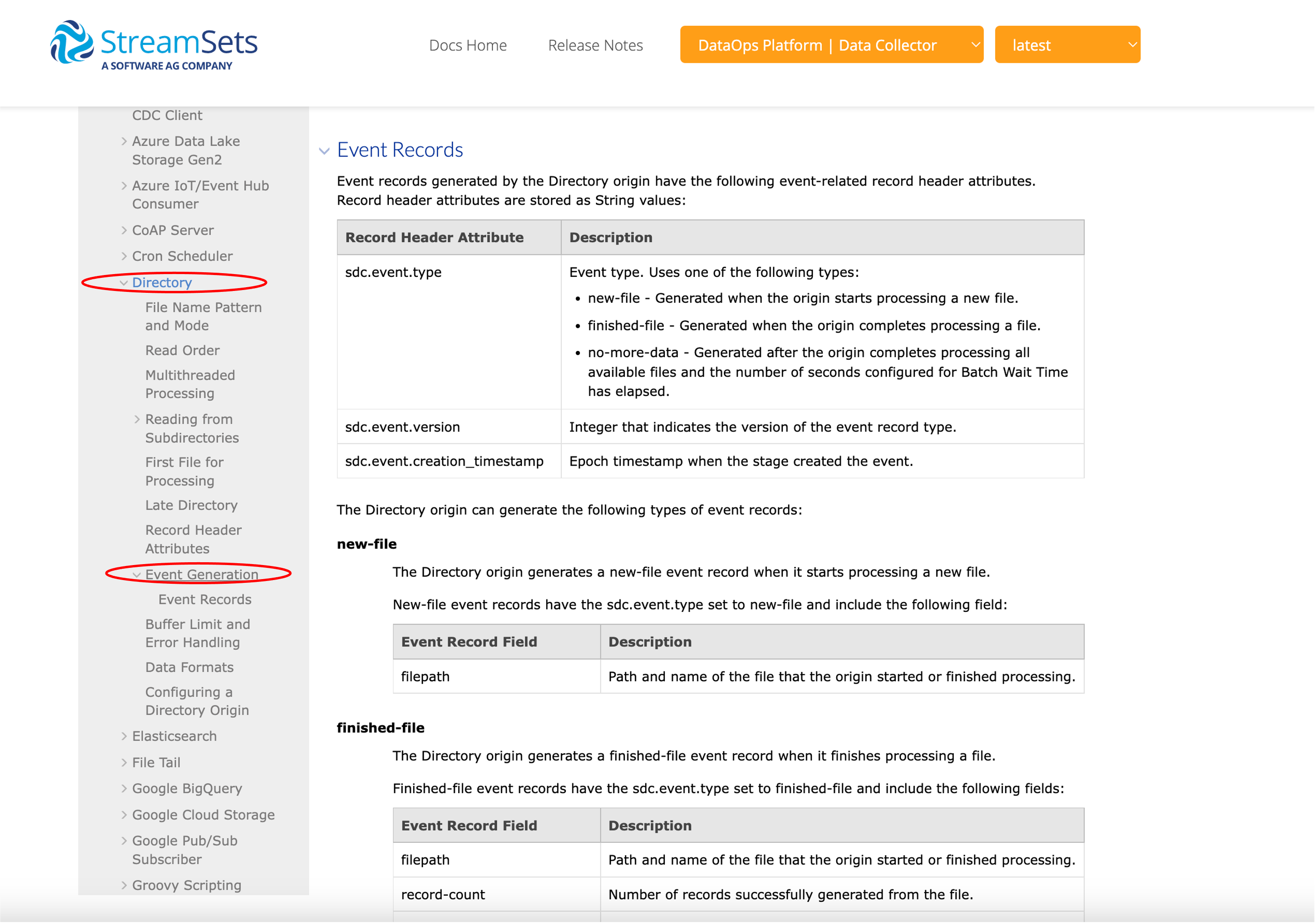The image displays a web page titled "Stream Sets." At the top, there's a distinctive, rounded triangular logo featuring bands of dark blue and mid-cyan blue hues. Adjacent to the logo, the text "Stream Sets" appears, with "Stream" in light blue and "Sets" in dark blue. Below, "a Software AG company" is written in dark blue.

On the left side, there is a comprehensive list of clickable areas and subcategories arranged in a vertical menu. The list begins with:
1. **CDC Client** 
2. **Azura, AZURE** 
3. **Data Lake, Storage Gen 2** 
4. **Azura IOT / Event Hub / Consumer**, each with a grey arrow indicating submenus.

Following these items, sections without arrows include:
5. **COAP Server**
6. **Cron Scheduler** 

Highlighted in a red oval with a down arrow is the item:
7. **Directory**

Additional sections without arrows include:
8. **Find Name**
9. **Pattern**
10. **Mode**
11. **Read Order**
12. **Multi-threaded Processing**

An item marked with a grey arrow is:
13. **Reading from Sub-directories**

Below it, further items are listed:
14. **First File for Processing**
15. **Late Directory**
16. **Recording Header Attributes**

Another highlighted section in a red oval features a drop-down arrow:
17. **Event Generation**

Following this is a list, alternating with items with and without grey arrows:
18. **Event Records**
19. **Buffer Limit and Error Handling**
20. **Data Formats**
21. **Configuration and Directory Origin**
22. **Elasticsearch** (with arrow)
23. **FileTail** (with arrow)
24. **Google BigQuery** (with arrow)
25. **Google Cloud Storage** (with arrow)
26. **Google Pub/Sub Subscriber** (with arrow)
27. **Groovy Scripting** (with arrow)

On the right-hand side, "Event Records" is written in blue. At the top of the page, there are three elements:
- **Docs Home**
- **Release Notes**

To the right, there is an orange rectangle labeled "Data Ops Platform" in bold white text, containing a line labeled "Data Collector" with a drop-down menu. Another orange rectangle labeled "Latest" in bold white text and containing a drop-down menu is positioned on the far right.

Under "Event Records," there are various headers, including:
- **CDC Event Type**
- **New File**
- **Finished File** in bold black text
- **Record Header Attribute**